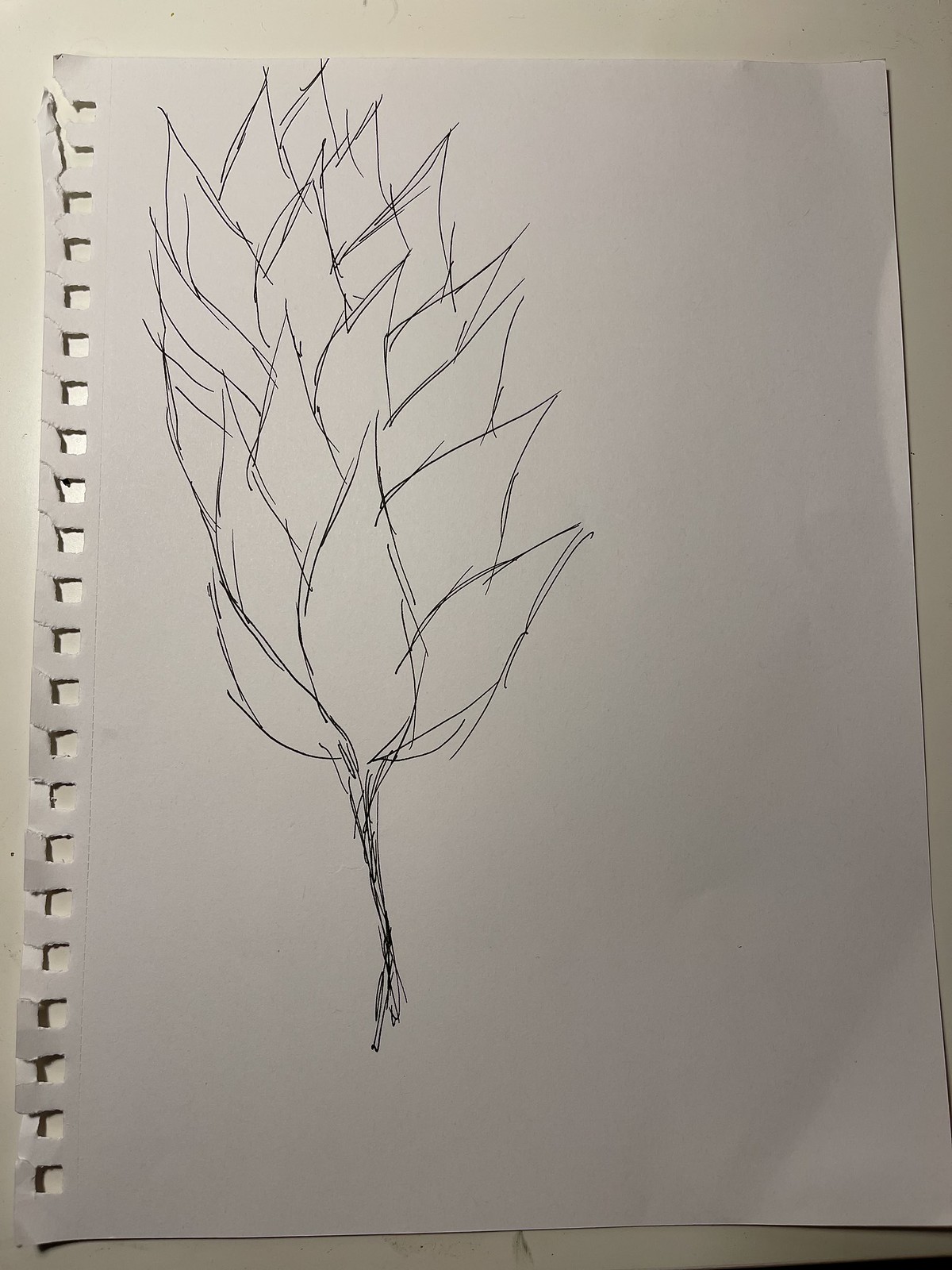This image captures a meticulously torn-out page from a drawing notebook, showcasing the perforated edge along the left side where it was removed. The pristine white sheet features a singular, detailed illustration of what appears to be a flower. The artistry, rendered in either pen or pencil, portrays a singular stem from which numerous petals elegantly branch out. Central to the composition are a series of overlapping leaves, extending upwards and diverging in various directions. Notably, the paper is immaculate, devoid of any other markings or blemishes, and rests on a plain, white countertop or desk, emphasizing the focus on the intricate floral drawing.